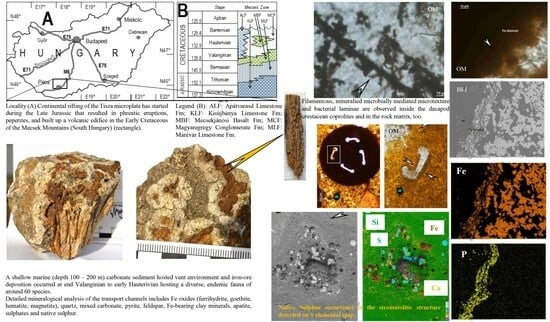The image resembles a detailed textbook page focusing on Hungary's geological features and mineral compositions from the Late Jurassic period. Dominating the top left is a black outline map of Hungary with annotations. Adjacent to the map is a legend explaining various elements like heights, weights, and depths. Below the map, two images of beige, brown, and gray rock formations are present, possibly depicting continental rifting effects. The left side includes detailed text discussing mineral deposits and geological microplates beneath Hungary, including notable areas like Budapest and information on the Cretaceous period depths. The right side features a grid of nine images highlighting different elevations and microbial presence in the rocks, indicated by the color differences—green, black, and white—with some marked as iron (Fe) and possibly potassium (P).